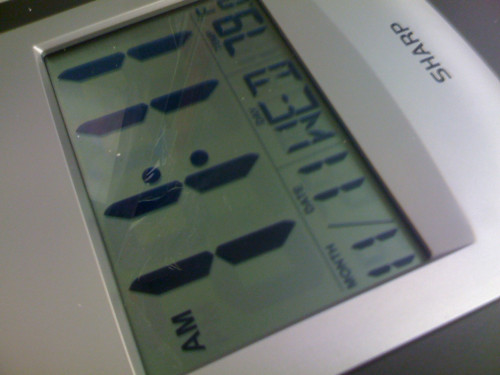This close-up photo features a rectangular digital atomic clock, manufactured by Sharp, set against a sleek silver background. The digital screen prominently displays the current time as 11:11 a.m. Below the time display, a row provides additional information, including the month as 11, the date as 11, and the day of the week as Wednesday, abbreviated as W-E-D. The temperature is shown as 79°F. The brand name "Sharp" is clearly inscribed on the bottom part of the clock's silver frame. The clock rests on a flat surface, emphasizing its modern, minimalist design.